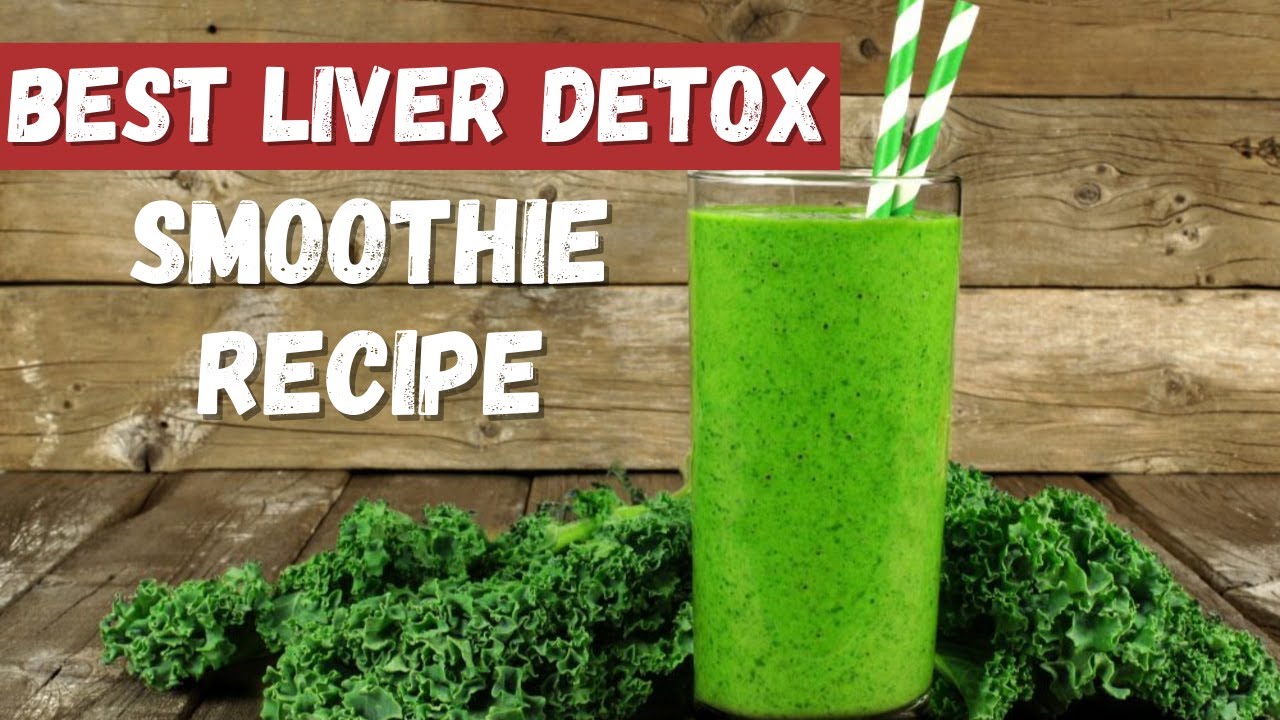In this detailed image, a green smoothie, speckled with black bits, fills a glass and sits prominently on a wooden surface, which appears to be part of a wooden deck or porch. The smoothie, garnished with two white and green striped straws leaning against the right side of the glass, is encircled by an assortment of green leaves, likely kale. The background features horizontal wooden slats, adding a rustic touch reminiscent of a barn wall. The setup places the smoothie slightly off-center to the right. In the upper left corner of the image, bold white block letters spell out "BEST LIVER DETOX" in all capital letters against a vibrant red rectangular background. Directly beneath, still in capitalized white block letters, the text reads "SMOOTHIE RECIPE." The color palette includes shades of green, brown, red, and white, emphasizing the natural and earthy theme of the photograph.